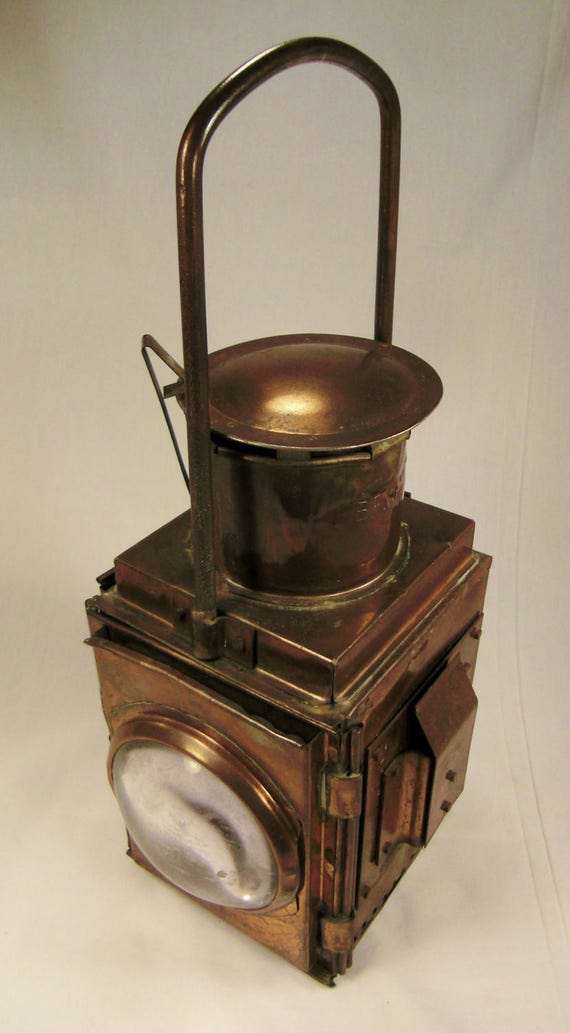The image features a vintage lantern, reminiscent of those used on ships or in lighthouses, placed against a beige background. The lantern has a distinctive bronze or copper hue, suggesting it might be made from these metals. Its design includes a lens on one side from which light was once emitted. The lantern’s structure comprises a box-like body with a handle on top for easy carrying or hanging. The upper part of the lantern has a round feature that resembles an ashtray. This antique piece evokes a sense of nostalgia, harking back to a time when such lanterns were essential tools for lighting.